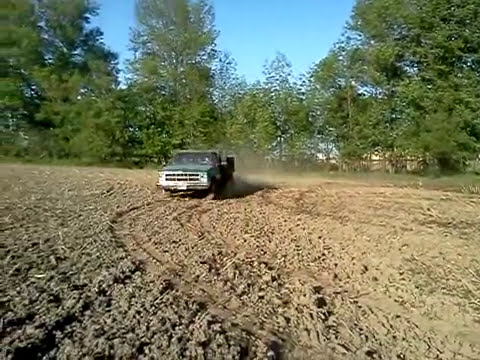This outdoor scene features a weathered, dark green pickup truck, potentially with a white grill, positioned slightly left of center and driving toward the camera across a dusty, brown dirt field. The field, which may have once held crops, now bears scattered tire tracks that loop and curve, leaving behind a light trail of dust and mud. These tracks create semi-circular patterns and indicate repeated passes over the land. Behind the truck, which appears dirty and dusty from its journey, stretches a grove of bright green deciduous trees occupying the upper half of the image. The trees form a dense backdrop with their tops cut off by the edge of the photograph, leading up to a clear, vivid blue sky without a single cloud. In the far distance, partially obscured by the trees, a building is faintly visible, adding another layer of detail to this serene, rural landscape.